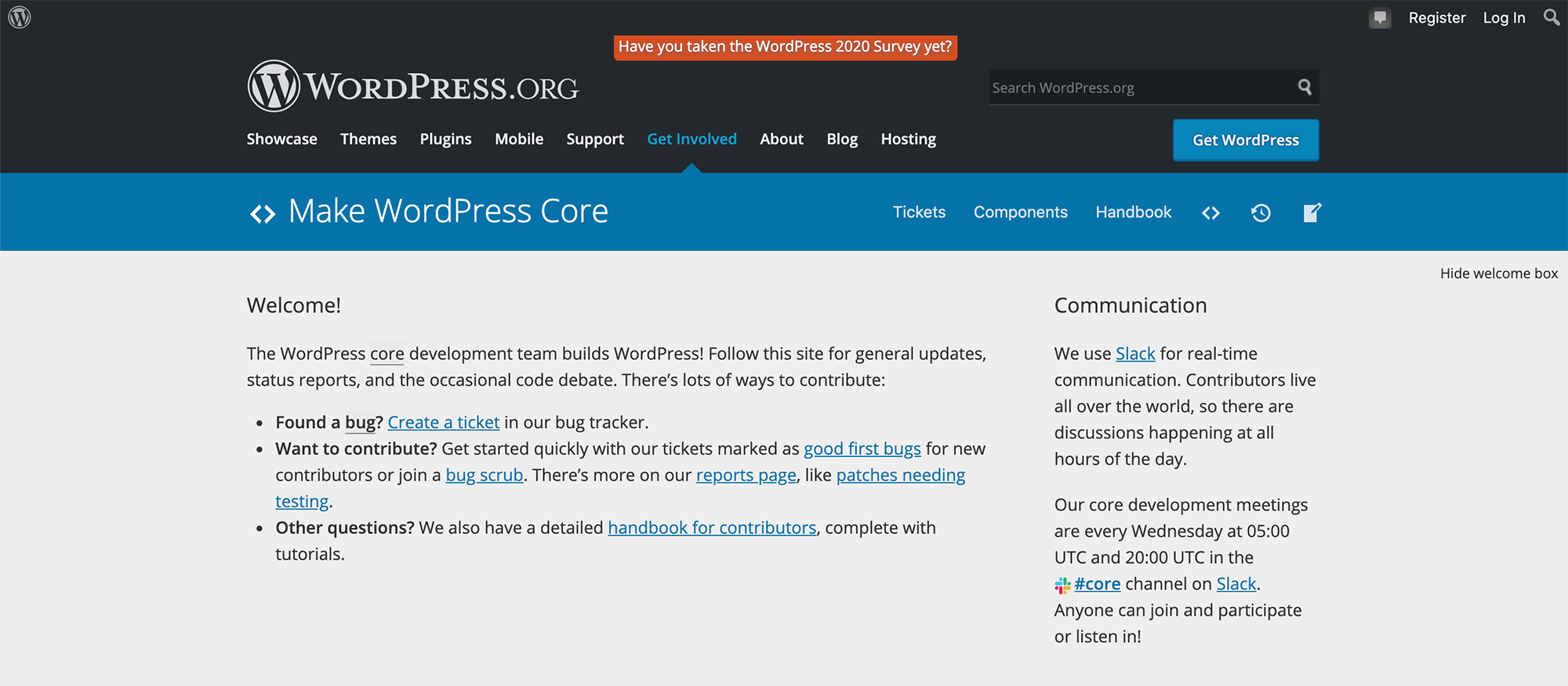Screenshot of the WordPress.org Landing Page

This is a screenshot of the landing page for WordPress.org, captured before any user has logged in or created an account. In the upper right corner, links for "Register" and "Log In" are visible, signaling that this is the homepage for new or yet-to-log-in users. Prominently placed at the center top is a red box with white text, urging users to participate in the "WordPress 2020 Survey."

The navigation bar features links for various sections: "Showcase," "Themes," "Plugins," "Mobile," "Support," "Get Involved," "About," "Blog," and "Hosting." The link for "Get Involved" is highlighted in blue, indicating that the current view is focused on this section. Below the navigation bar, there's a blue band that says "Make WordPress Core," which includes links to "Tickets," "Components," and "Handbook."

The upper part, comprising the navigation and title sections, takes up approximately the top 30% of the image. The remaining 70% is dominated by text content. The left side, which occupies about 50% of the screen, contains a welcome message: "Welcome, the WordPress core development team builds WordPress. Follow the site for general updates, status reports, and the occasional code debate. There are lots of ways to contribute," followed by three bullet points listing various ways to get involved.

The right-hand column, taking up roughly 30% of the screen, is headed with "Communication" and informs users that "We use Slack for real-time communication."